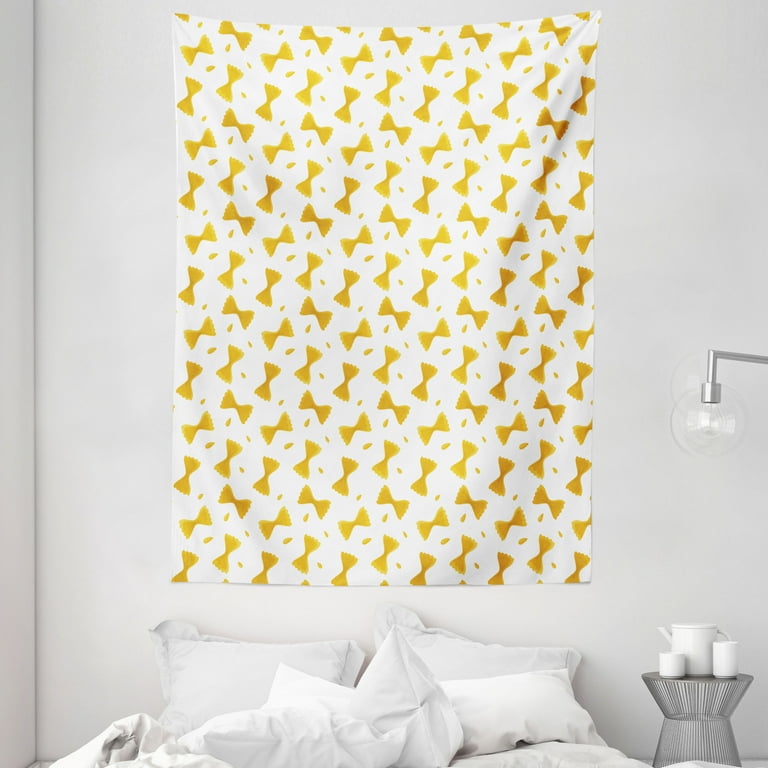The image depicts a cozy bedroom with plain white walls, adorned by a prominent rectangular cloth hanging on the wall, which measures approximately five by four feet. The cloth, slightly wrinkled at the upper right-hand corner, features a repetitive pattern of yellow bow tie shapes, reminiscent of pasta, set against a white background. Below the hanging fabric, the bed is unmade with white bed sheets, pillowcases, and a crumpled blanket, along with pillows strewn about casually. To the right of the bed, there is a minimalist nightstand constructed from metal rods with a flat top, holding a small white ceramic tea set consisting of two cups and a pot. Adjacent to the nightstand, a wall-mounted lamp with a chrome arm and a solid, round glass globe illuminates the area, adding a sleek modern touch to the serene, slightly disheveled space.